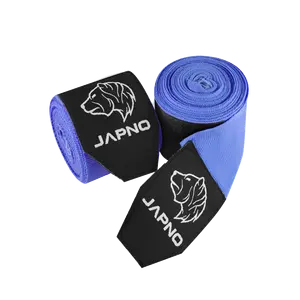The image displays a color photograph of two tightly coiled straps, resembling the color of doctor's scrubs—a purplish blue hue. Each strap is partially unraveled, revealing a black label at the end bearing the text "JAPNO," noticeably stylized with the letter "A" as an upside-down V. The labels also feature a white outline of a lion or wolf head, adding a subtle, stylized animal motif. One of the coiled straps is positioned to show its cylindrical shape, while the other lies flat, showcasing its rounded coils. The straps appear to be made of a thin, flexible fabric, possibly cotton, suitable for gymnasium or athletic use. The robust nature of the logo tab suggests it might be used for gripping or tightening.